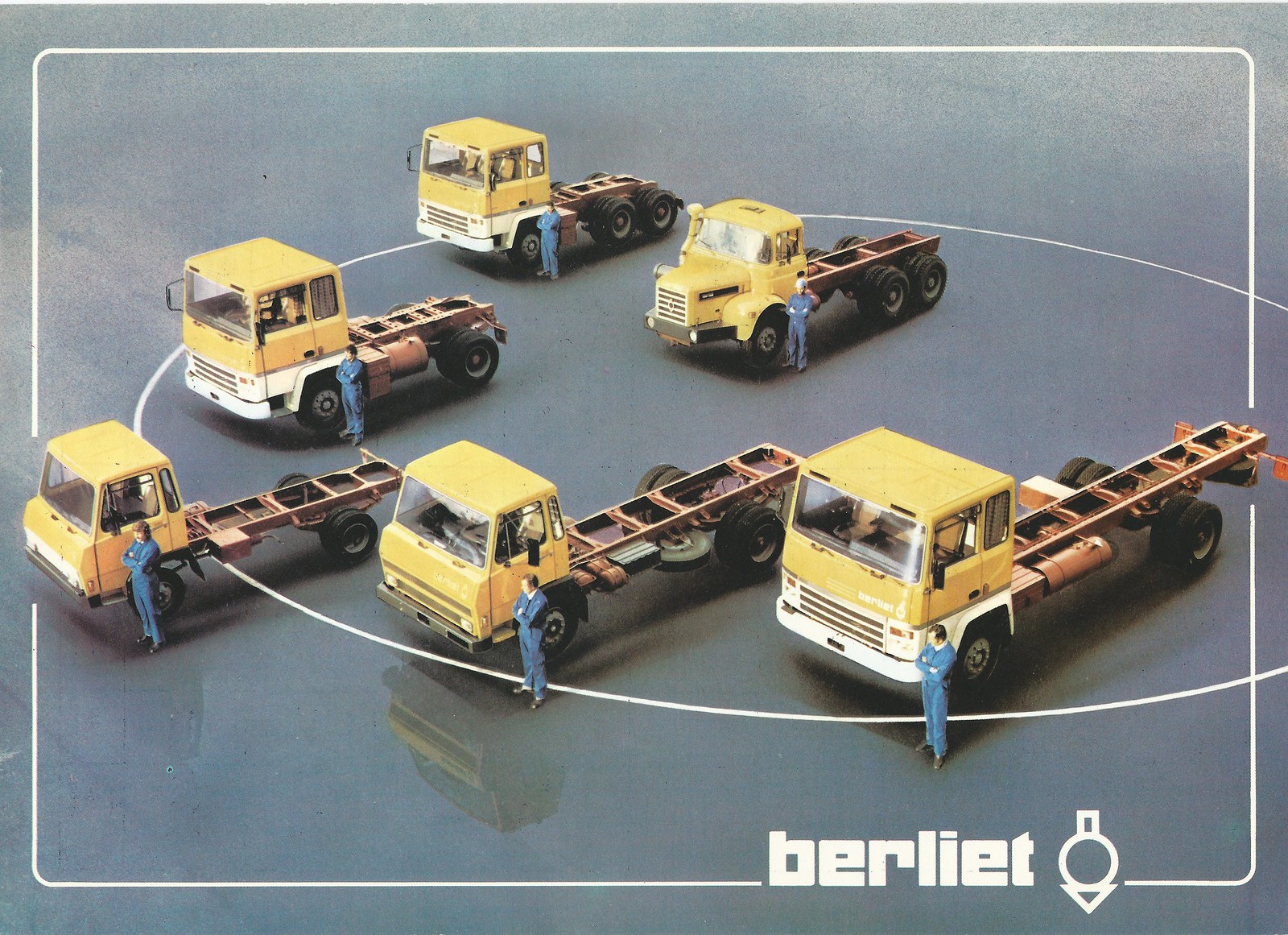The image portrays an overhead view of six flatbed trucks with a distinctive vintage design, each featuring a yellow cab and a narrow flatbed. Five of the trucks are of the same length, while one is noticeably longer. Each truck is accompanied by a worker in blue attire standing next to the driver's side door with arms crossed. The background has a glossy, reflective gray surface, highlighting the reflections of the trucks and creating a visually appealing effect. The scene is framed with a white border incorporating rounded corners. At the bottom of the image, the text "BERLIET" is displayed in white, accompanied by a unique logo consisting of an upside-down triangle, a circle on top, and a small rectangle above the circle. This setup suggests the image could be part of an advertisement for Berliet vehicles.